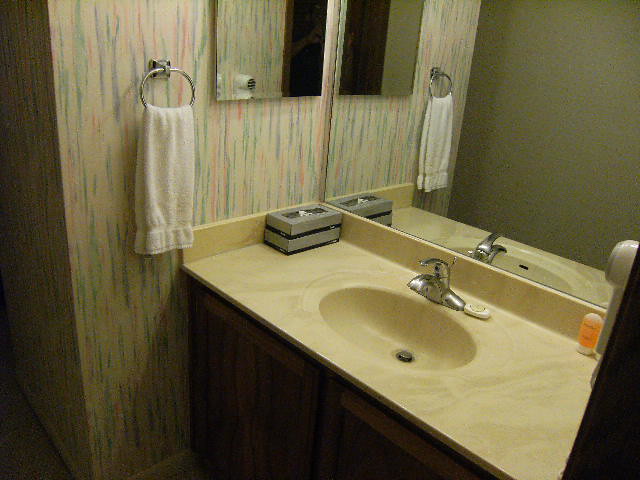This detailed photograph showcases the interior of a bathroom, perfectly framed in a rectangle. The most striking feature is the mirror, which reflects an exact image of the bathroom, creating an intriguing visual symmetry. 

The left wall, extending from the top left corner to the bottom, is adorned with light cream wallpaper, accented by delicate vertical streaks of light blue, green, pink, and red. A silver oval towel holder is mounted on this wall, holding a neatly hung white terrycloth towel with visible edges at the bottom.

In the upper right corner of this left wall, a clear decoration with a brown stripe adds a touch of elegance, though its exact nature is ambiguous. 

Beneath this setup lies the bathroom sink, featuring a cream marbleized pattern. The silver faucet gleams next to a silver drain at the center of the sink. Beside the faucet is a small white ceramic item with a green centerpiece.

Moving to the right side of the image, a container with orange and white elements is situated. Below it rests a Kleenex box, and attached to the wall is a hair dryer, suggesting this is likely a hotel bathroom, as such fixtures are common in such settings.

The mirror, positioned from the top center to the upper right corner, reflects not only the wall-mounted decoration and towel holder but also the Kleenex box, sink, faucet, and an olive green wall behind the camera, enriching the photograph with depth and detail.